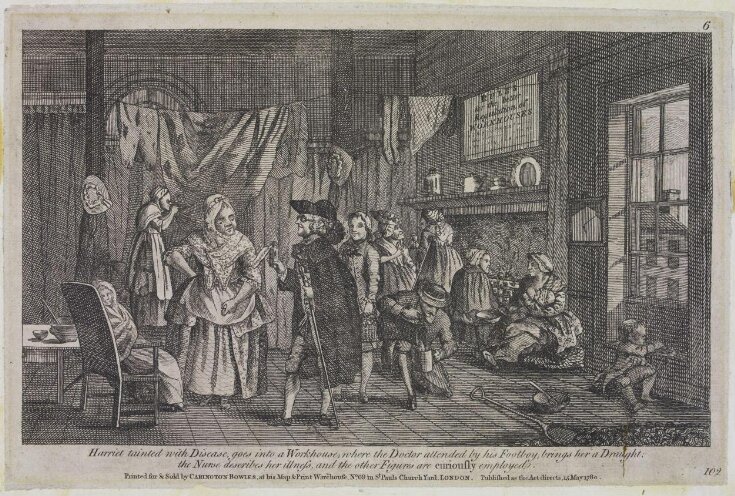An intricate black-and-white drawing, reminiscent of 18th to 19th century illustrations, depicts a bustling room inside a workhouse. The room is filled with various characters, all dressed in period clothing. At the heart of the scene stands an elderly woman in a white dress, accompanied by a well-dressed doctor in a long coat, wig, and black hat. He is attended by a foot boy and presents the woman with either medicine or a piece of paper. The woman, looking frail and wrapped in blankets, is described as Harriet, tainted with disease. Nearby, a nurse explains Harriet's condition to the doctor.

The room is detailed with a large fireplace adorned with a sign that reads "Rules of the Workhouse," and a clothesline strung overhead with items hanging to dry. A child sits in the foreground near a window, which reveals a building outside. The background is filled with other figures, including women and children, engaged in various activities, creating a lively, yet somber atmosphere. Below the image, in tiny script, an inscription provides contextual details and mentions the printing origins, though much of this text is hard to read. The sketch utilizes cross-hatching for shading, adding depth and texture to the scene, and the numeral "102" is noted in one corner.